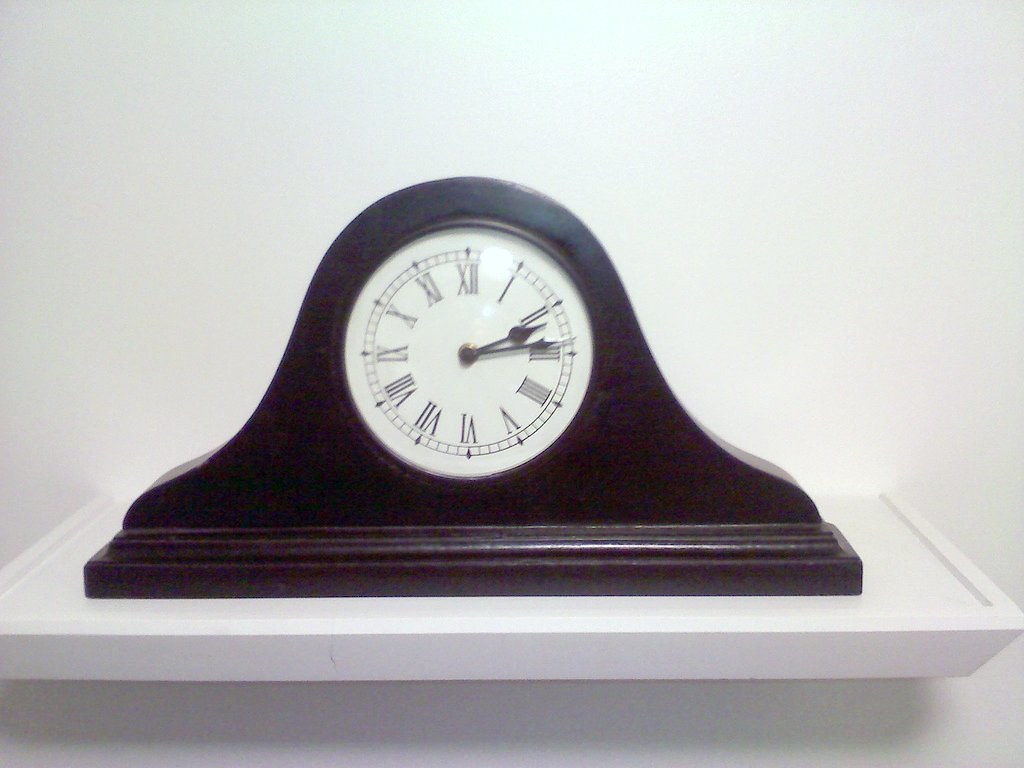This is a horizontal color photograph of a classic brown wooden mantelpiece clock with a white face, black Roman numerals, and decorative black hands indicating 14 minutes past 2. The clock is housed in a curved, bell-shaped frame that has a wide, shiny base and rounded edges extending upward like a hill. A gold pin connects the hands at the center of the clock face, adding a subtle accent. The clock is situated on a pristine white shelf against a white wall, with light reflecting off the glass surface covering the clock face.